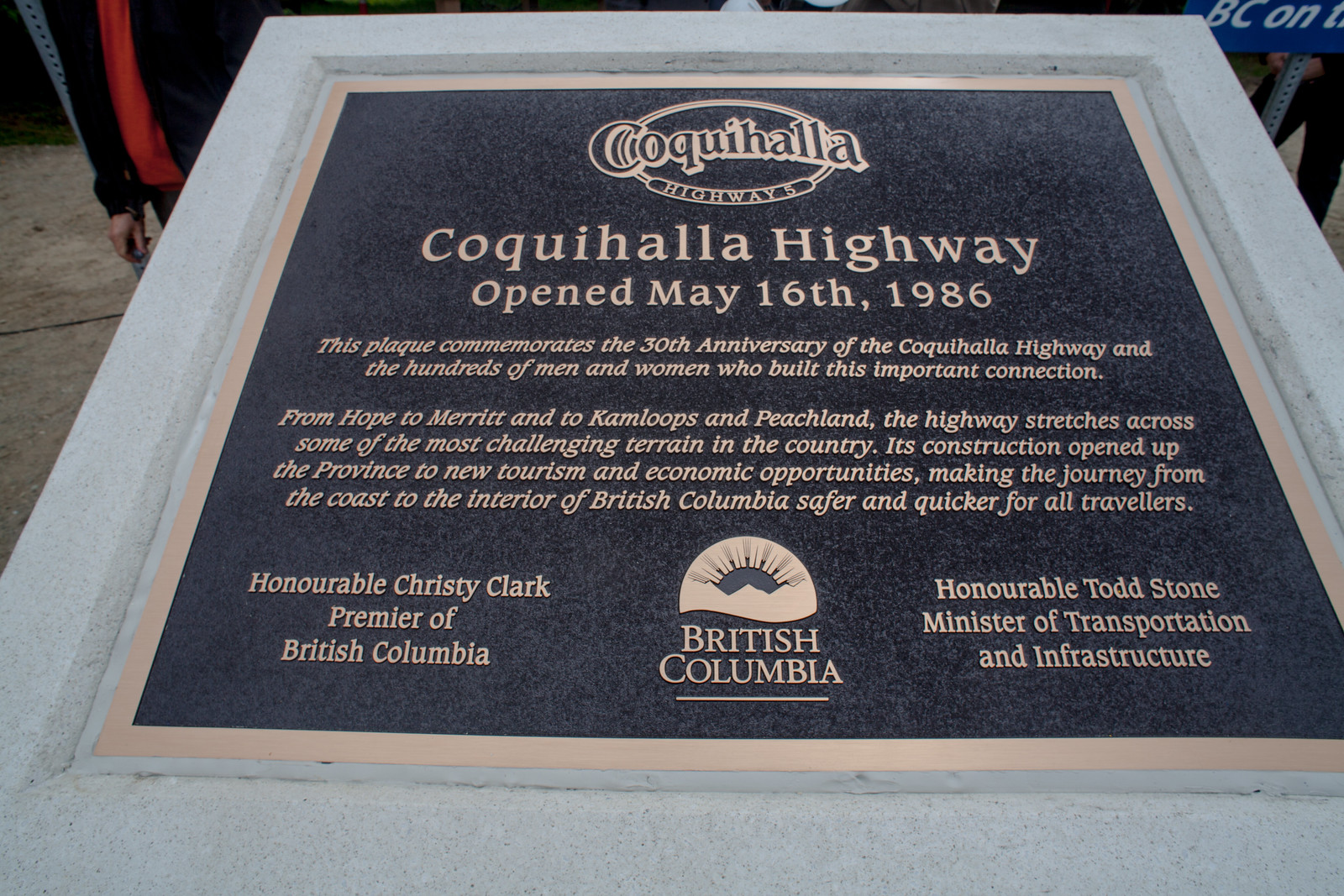This outdoor commemorative plaque, set in a gray pedestal-like frame, celebrates the Coquihalla Highway, which opened on May 16, 1986. The plaque has gold-lined, gold writing on a black background and features a circle icon with "COQUIHALLA HIGHWAYS" and "Coquihalla Highway opened May 16, 1986." It commemorates the 30th anniversary of the highway and honors the hundreds of men and women who built this crucial connection. Stretching from Hope to Merritt, Kamloops, and Peachland, it traverses some of Canada’s most challenging terrain. The construction of this highway revolutionized travel, making the journey from the coast to the interior of British Columbia safer and quicker, while opening the province to new tourism and economic opportunities. The bottom of the plaque bears the British Columbia logo, along with the names of the Premier and the Minister of Transportation for British Columbia.